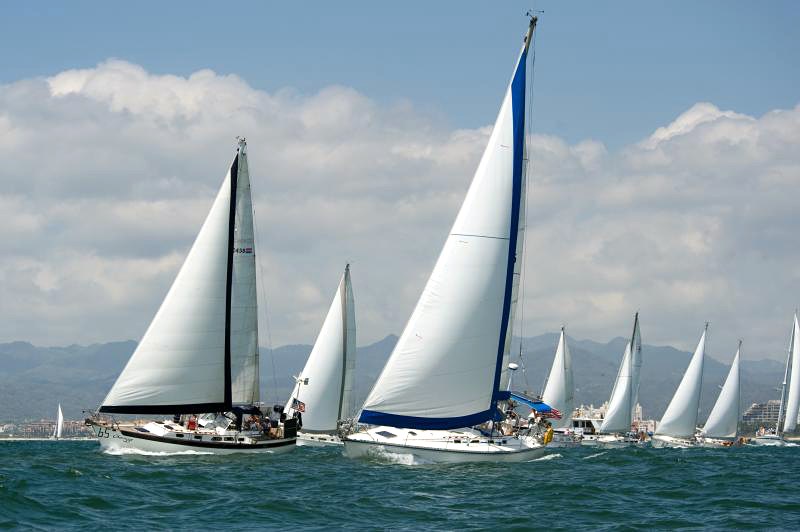The photograph, horizontally oriented and rectangular in shape, captures a serene ocean scene on a bright summer day, with the image likely taken from another watercraft. Multiple sailboats glide gracefully across the calm, blue-green waters, participating in what appears to be a sailing regatta. The two prominent sailboats in the foreground boast distinct sails—one with a blue stripe and another with a black stripe—while a number of smaller sailboats with white sails can be seen further back. The background is adorned with layers of mountainous terrain stretching from left to right, providing a picturesque backdrop. The sky above is dotted with fluffy white clouds and patches of clear blue sky, adding to the beauty of this tranquil setting. A slight haze, possibly from pollution, creates a dreamy effect. In the bottom right corner, a large building can be seen on the distant shoreline, adding a touch of human presence to the otherwise natural scene. Overall, the photograph vividly captures the essence of a peaceful and competitive summer day on the ocean.